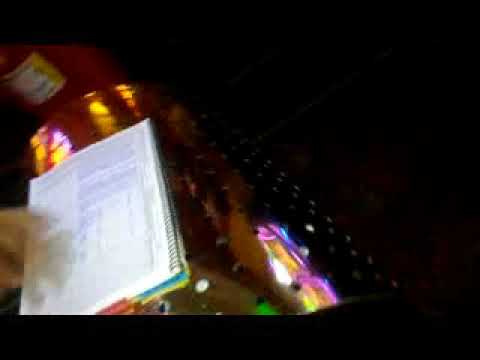The image depicts a slightly tilted spiral notebook with silver rings and white pages, held by a hand emerging from the left side. The notebook is detailed with blue, yellow, and red tabs, and is secured by a red clip. While the paper has blue writing, the text is illegible due to the overall blurriness of the photo. The setting appears to be a dark environment, potentially a bar or nightclub, suggested by the colorful strobe-like lights in the background mingling in hues of yellow, pink, red, blue, and white. Additional elements in the photo include what seems to be the bottom of a beverage bottle in the upper left corner, possibly hinting at a social setting. The bottom of the image features solid black, and one can faintly discern what might be a forehead and hairline of a person at the lower center. The image conveys a vibrant yet out-of-focus atmosphere, with a large red object, possibly furniture, slightly discernible behind the notebook.